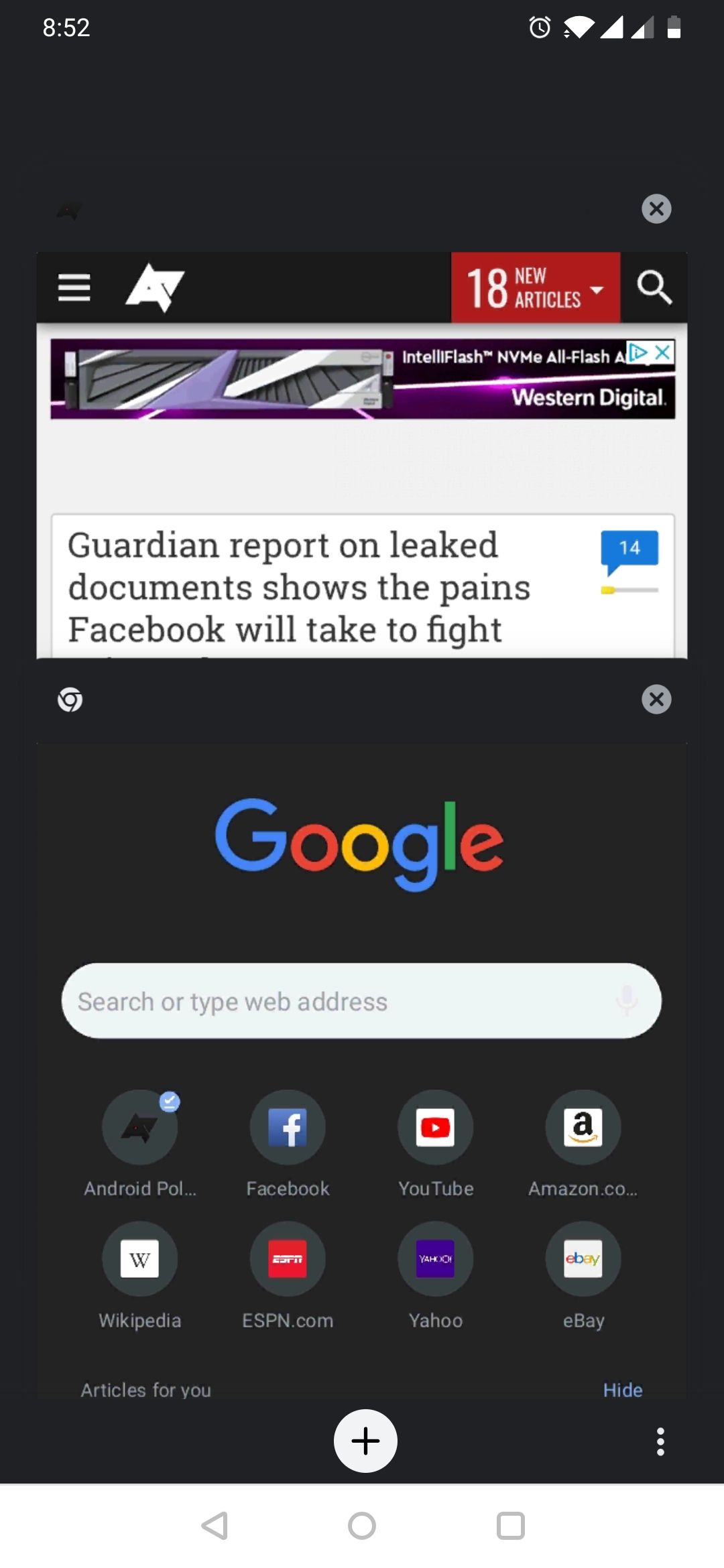This image is a screenshot of a mobile phone's homepage, specifically within the Google app interface in night mode, characterized by a dark gray background. 

**Top Section:**
- **Time:** Displayed prominently at the top center of the screen.
- **Icons:**
  - Top left: Alarm clock icon.
  - Top right: Wi-Fi signal, data signal, and battery icons.

**Middle Section:**
- **Banner Ad:** Positioned above the Google logo, featuring a rectangular advertisement banner. The banner includes a headline from The Guardian about Facebook's efforts in response to leaked documents. A small "X" button is located in the top right corner of this ad, allowing users to close it.
- **Google Logo:** Located centrally beneath the banner ad.

**Search Bar:**
- Below the Google logo is a long search bar with grayed-out text that says "Search or type web address."

**Icon Row:**
- **Website Suggestions:** Four circular icons are displayed:
  - Android
  - Facebook
  - YouTube
  - Amazon

**Bottom Section:**
- **Additional Icons:** Other icons represent eBay, Yahoo, Wikipedia, and ESPN.
- **Articles for You:** Text on the bottom left suggests personalized content.
- **Plus Sign:** A circular plus sign is centered at the bottom, likely for adding new pages or tabs.
- **Menu Bar:**
  - Bottom left: A triangle icon pointing to the left (back button).
  - Bottom center: A circle (home button).
  - Bottom right: A square (recent apps or multitasking).

This detailed interface screenshot highlights the user's typical engagement with the Google app, integrated within the cohesive design of a mobile device's night mode.